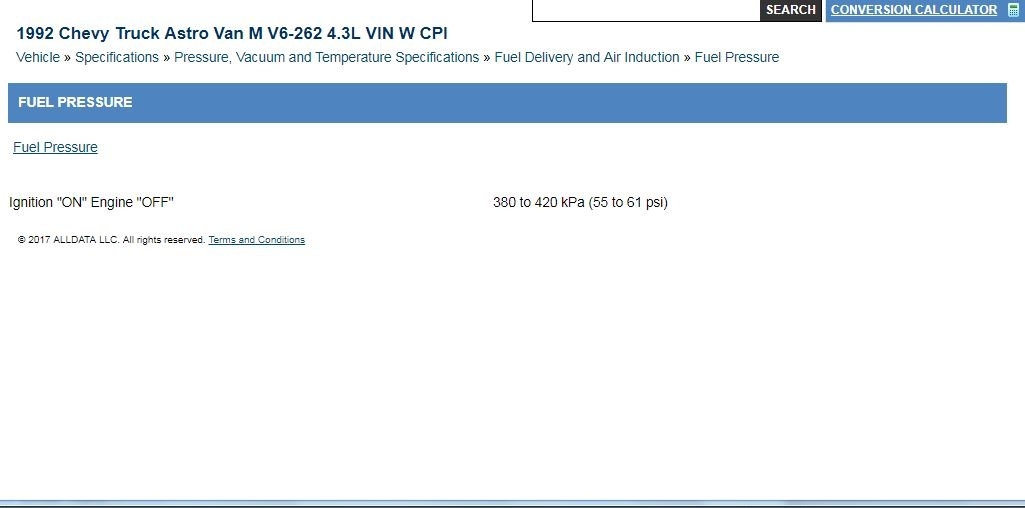The image displays the interface of a detailed automotive website. At the very top right corner, there's a search bar for entering keywords to initiate a search. Adjacent to the search bar is a conversion calculator link, identifiable by a small sketch of a calculator.

Below this top section, a bolded, grey heading on the left reads: "1992 Chevy Truck Astrovan M V6-262 4.3 litre VIN WCPI." This indicates that the information pertains to this specific vehicle model. The context of this information is clarified as it originates from various sections on the website, namely: Vehicle Specifications, Pressure, Vacuum and Temperature Specifications, Fuel Delivery and Air Induction, and specifically Fuel Pressure.

A blue banner spans the screen underneath the heading, with "FUEL PRESSURE" prominently displayed in white capital letters on the left side. Beneath this banner is another "Fuel Pressure" text presented as a clickable hyperlink. Below this link, it specifies instructions and measurements: "Ignition on, Engine off" and "380-420 kPa (55-61 PSI)."

At the very bottom, a copyright notice states: "© 2017 ALLDATA LLC All Rights Reserved," accompanied by a blue 'Terms and Conditions' hyperlink.